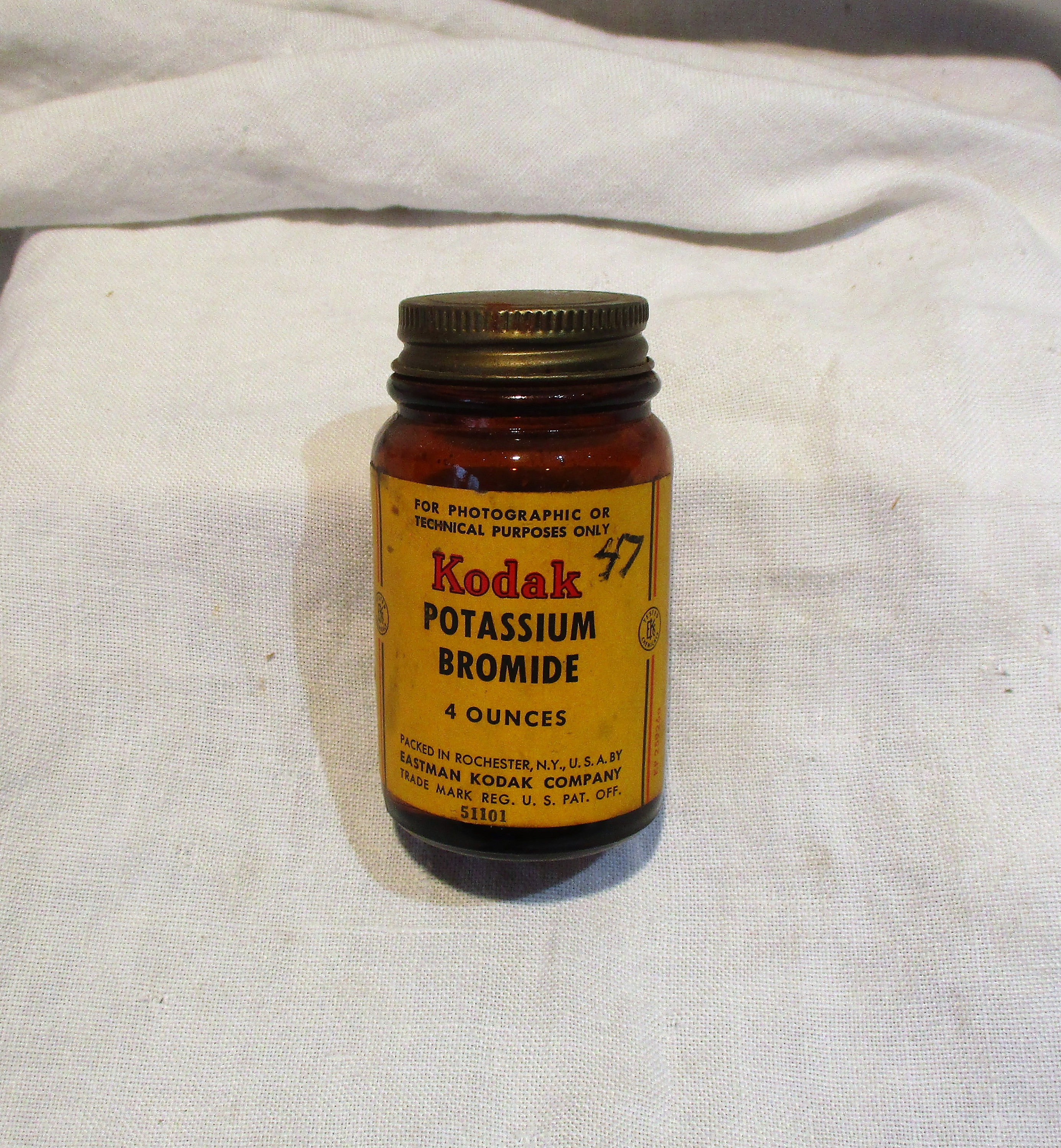The image features a vintage glass jar of potassium bromide designed for developing film, reminiscent of a mason jar or a jar of spaghetti sauce. It is topped with a screw-on, goldish tin lid that shows signs of age with visible rust. The jar is adorned with a bright yellow label. Prominently, the label bears the red Kodak logo and the number "47" inscribed on the upper right. Below this, black text reads "for photographic or technical purposes only," followed by "potassium bromide," and the quantity "four ounces." At the bottom of the label, it states "packed in Rochester, New York, USA, by Eastman Kodak Company." The jar is placed on a white cotton cloth, which is slightly folded near the top, revealing some fabric imperfections and casting a shadow of the jar. Subtle gray tones appear in the background.